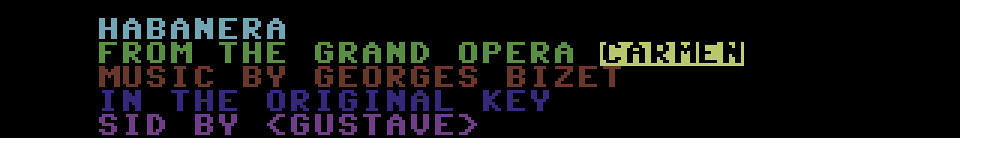This image is a horizontally-oriented screenshot featuring text styled in the aesthetic of classic Atari video games. The title "Habanera" is prominently displayed at the top in bold blue lettering. Beneath it, "From the Grand Opera" is written in vivid green. The name "Carmen" stands out in black text highlighted with a yellow hue. Below this, in a rich auburn color, the image credits "Music by Georges Bizet." The phrase "In the Original Key" appears in a dark purple tone. Lastly, at the bottom, in light purple text framed by brackets, the image reads "Sid by Gustav." The image is devoid of additional graphics or details, focusing solely on the text elements presented in retro video game-like fonts.